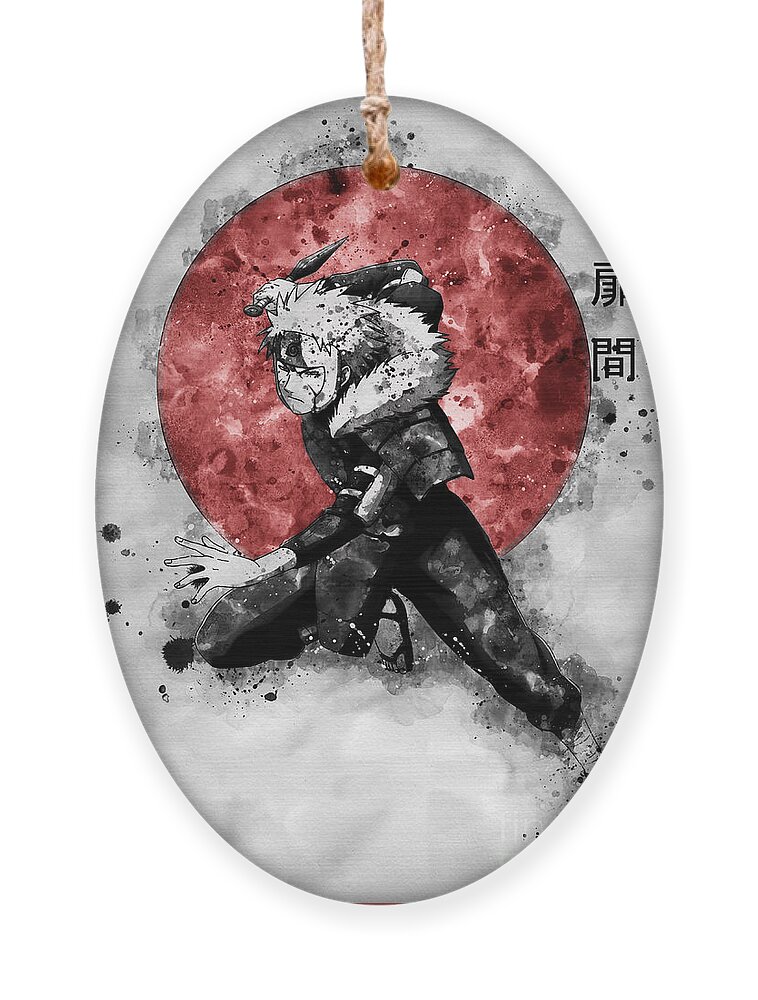This image depicts an oval-shaped ceramic medallion or pendant with a light brown string threaded through a hole at the top for hanging. At the center of the medallion is a dynamic black and white illustration of an anime-style ninja character with long, spiky hair and a headband that covers his forehead and cheeks. The ninja, dressed in a fur-trimmed, oversized jacket with shoulder pads, long pants, and sandals, is captured in a crouched, aggressive stance. His right knee is bent with his leg dug into the ground, while his left leg is stretched to the side. He holds a small, cloth-wrapped dagger behind him in his right hand, poised for attack, and extends his left hand forward. Behind him, there is a prominent red circle, reminiscent of the Japanese flag, with artistic black and white splotches within it. Scattered throughout the medallion and below the character's extended hand are additional black ink blots and black and white dots, adding to the artistic effect. On the midsection of the right side of the medallion, there are Japanese characters inscribed in black. The entire scene is rendered in a grayscale palette, with the striking exception of the vivid red circle.